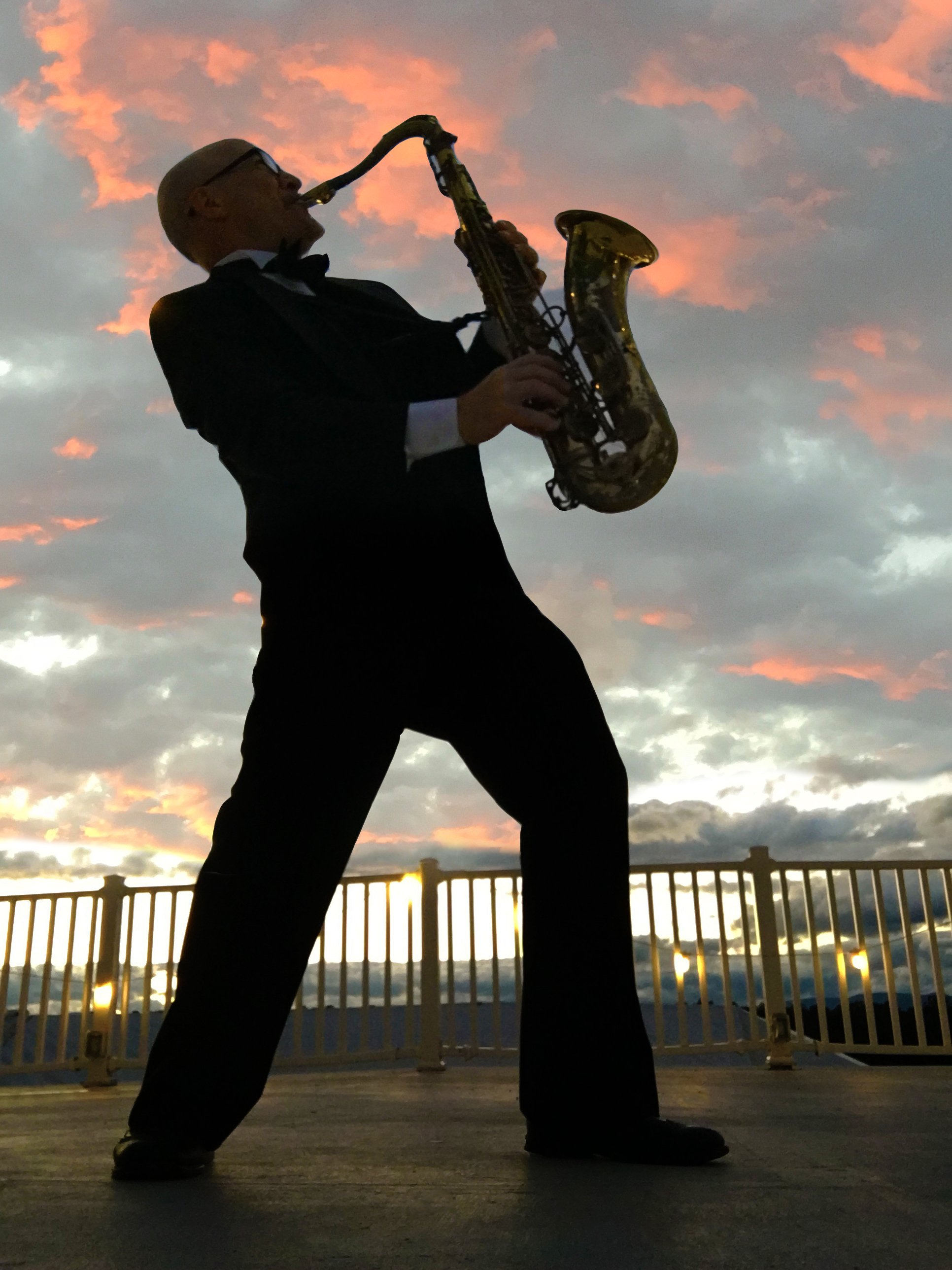Against a backdrop of a stunning sunset sky filled with clouds tinged with bright pink, peach, orange, and gray hues, a man stands on a flat, concrete-style wooden deck, leaning back slightly as he passionately plays his saxophone. Dressed elegantly in a tuxedo, the bald-headed man, adorned with glasses, is captured in a dramatic silhouette, emphasizing his posture and the raised saxophone pointing towards the upper right. The deck is bordered by a metal railing that glistens in the fading light, positioning the saxophonist almost in profile as he faces to the right, creating a striking contrast against the vibrant colors of the twilight sky.